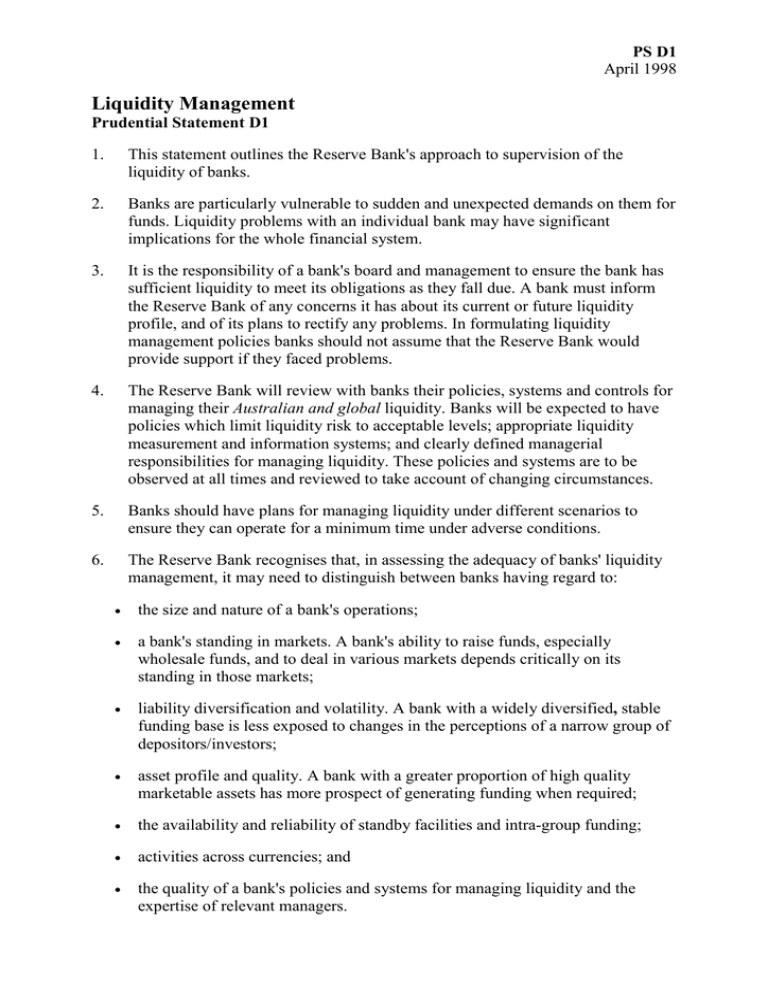The document displayed is a white page resembling a word document, filled with numerous paragraphs of text. At the top, it is titled "Liquidity Management – Prudential Statement D1," with the upper right corner marked "PSD1, April 1998."

This statement outlines the Reserve Bank's approach to the supervision of bank liquidity. It underscores the vulnerability of banks to sudden and unexpected demands for funds, highlighting how liquidity issues in one bank can impact the entire financial system. Therefore, it is the bank's board and management's responsibility to ensure sufficient liquidity to meet their obligations as they arise.

Banks are required to inform the Reserve Bank of any concerns regarding their current or future liquidity profiles, alongside their plans to address any issues. When formulating liquidity management policies, banks should not assume the Reserve Bank will provide support during liquidity problems.

The Reserve Bank will review banks' policies, systems, and controls concerning both their Australian and global liquidity. Banks must maintain policies limiting liquidity risks to acceptable levels, have proper liquidity measurement systems, information systems, and clearly defined managerial responsibilities for liquidity management. These policies must be observed continuously and adapted to changing circumstances.

Moreover, banks should have contingency plans for different liquidity scenarios to ensure continued operations during adverse conditions. The Reserve Bank may need to differentiate between banks by considering factors such as the size and nature of operations, market standing, liability diversification and volatility, asset profile and quality, reliability of standby facilities, funding activities across currencies, and the quality of policies and management expertise regarding liquidity.

In essence, the document elaborates on how liquidity management functions within the financial system and outlines the expectations from banks to ensure their liquidity practices are robust and effective.